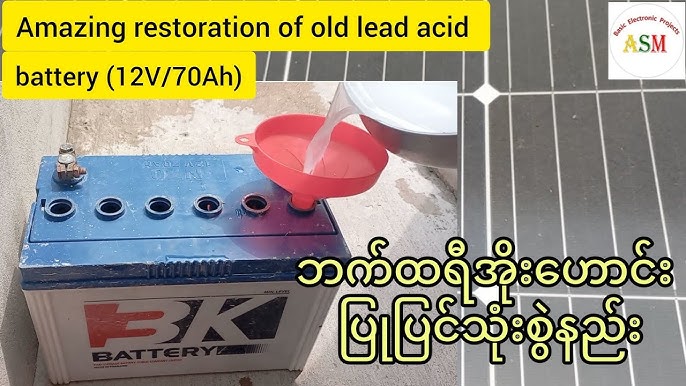The image depicts a detailed scene focused on the restoration of an old lead-acid car battery, specifically labeled as a 3K battery. The battery, primarily colored in white with a blue top, features six holes, one of which is currently being refilled with a white liquid through a red funnel. The upper left corner of the image, set against a yellow background, prominently displays the text, "Amazing Restoration of Old Lead Acid Battery (12V-70AH)." Adjacent to the battery image is a textual overlay: "Basic Electronic Projects ASM." This logo, situated in the upper right corner, uses a combination of red, yellow, and green lettering on a white background. The overall backdrop of the image resembles a dark gray tile grid pattern. Additionally, foreign script, possibly from the Indian subcontinent, is visible in the bottom right corner of the image, adding an element of non-Latin characters to the scene. The composition and details suggest the image could be a screenshot from a YouTube video tutorial on battery restoration.